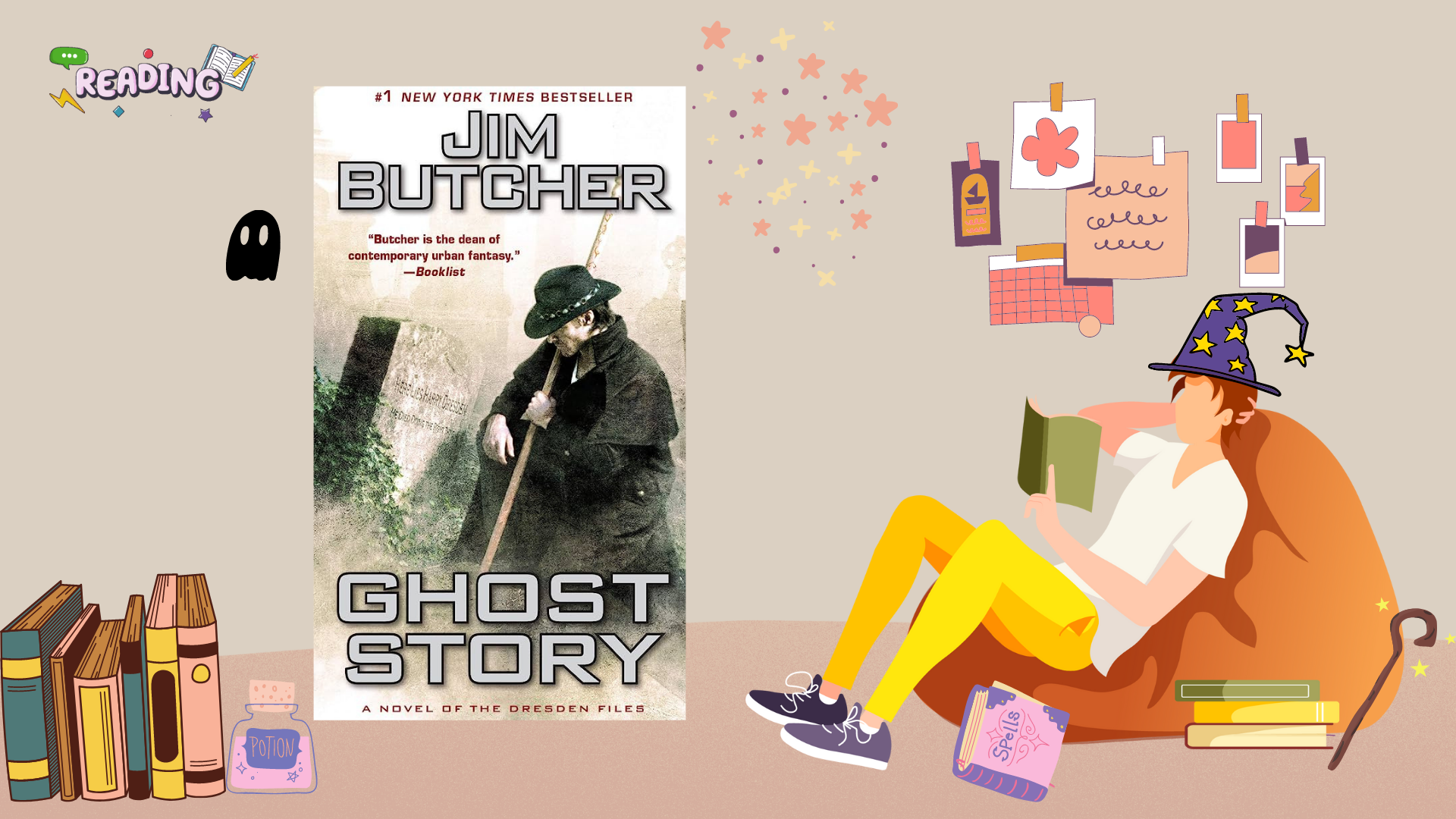In this horizontally-oriented rectangular image, we are presented with a visually engaging combination of advertisement and artwork. The backdrop features a whimsical, cartoon-like illustration. 

In the lower right corner, an orange beanbag chair is prominently displayed. Seated on it, facing west, is a young person adorned in a blue wizard hat decorated with yellow stars, deeply engrossed in reading a book. Above this young reader, papers are haphazardly attached to a wall, adding to the scene's charm.

On the lower left side of the image, colorful illustrations of books are neatly stacked against one another, creating a vivid and inviting atmosphere. Meanwhile, in the upper left corner, the image reads "Reading" in bold, block-style lettering.

The central focus of the image is a book cover, featuring an illustration of a man wearing a cape and a cowboy-style hat, looking downward. This cover bears the title "Number One New York Times Bestseller, Jim Butcher, Ghost Story: A Novel of the Dresden Files," highlighting the book’s acclaim and author.